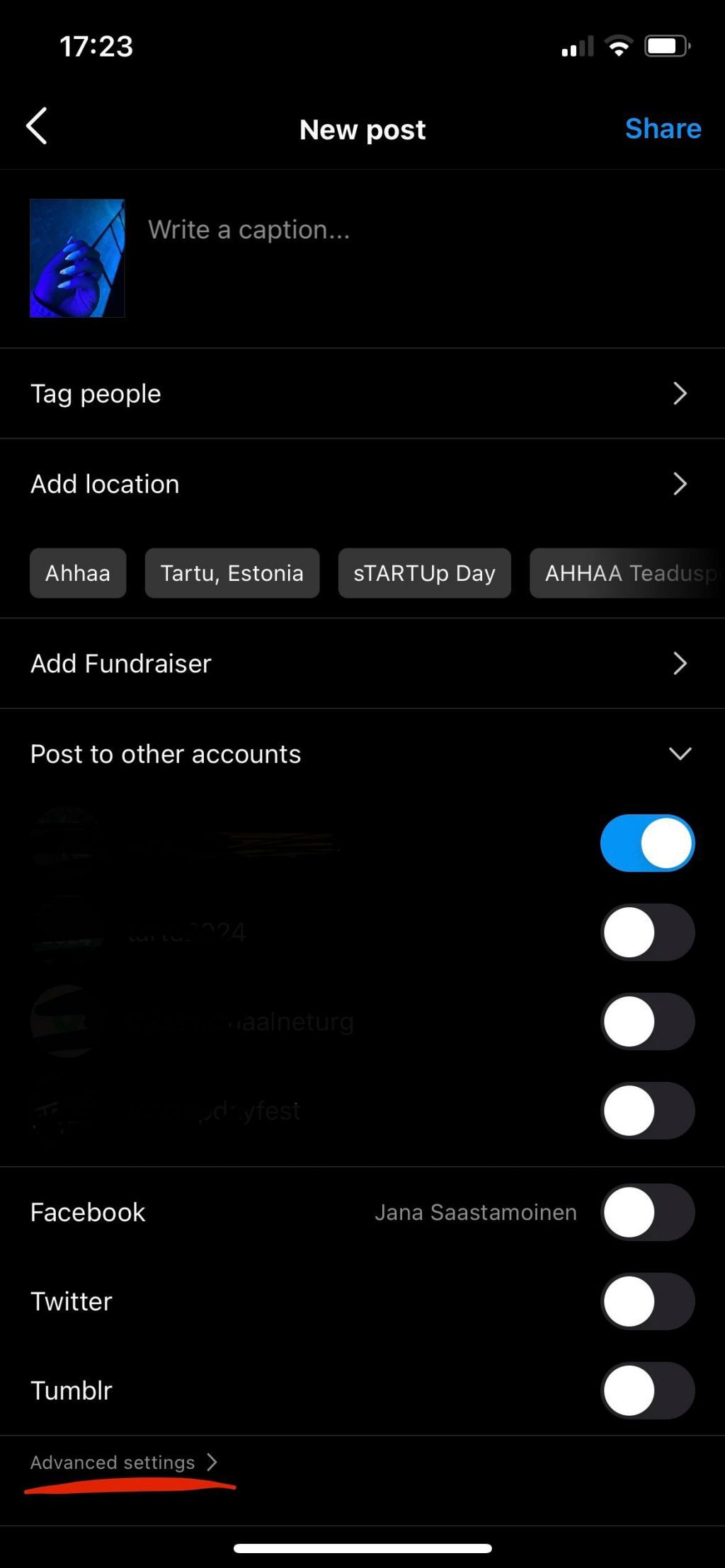The screenshot showcases a mobile phone interface at 5:23 p.m., as indicated by the time display at the top. The status bar reveals the strength of both Wi-Fi and cellular signals, alongside a battery life nearing 80%. Below, the screen focuses on a social media platform where the user is in the process of creating a new post. The image intended for posting features a hand against a vivid blue background. No caption has been added yet, nor have any people been tagged or a location specified. The user has the capability to add a fundraiser, although this option remains unselected. However, they have opted to cross-post the update to other social networks, including Facebook, Twitter, and Tumblr. At the bottom, an "Advanced Settings" link is highlighted in red, indicating instructional emphasis on navigating these options.